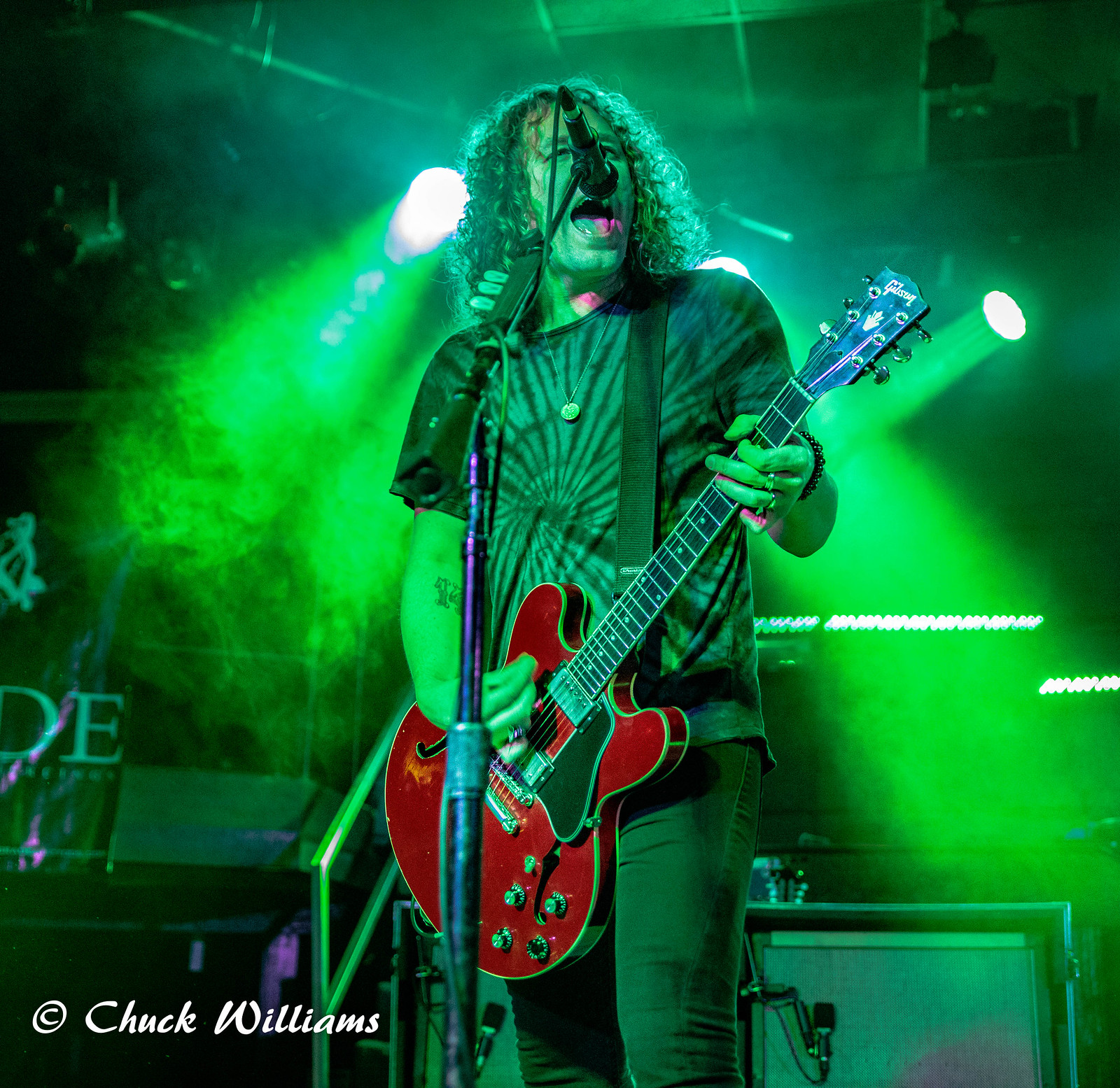In this perfectly square image, a male musician with curly shoulder-length hair stands on a stage, passionately singing into a microphone while playing a red and black electric guitar. He is dressed in a black tie-dye shirt and jeans. His right forearm features a visible tattoo, and he accessorizes with multiple rings on his left hand, a black beaded bracelet, and a necklace. His mouth is open mid-performance, capturing his intensity. The image has an overall green hue, with stage lighting and smoke creating a dramatic backdrop. Amplifiers and additional stage lights are visible behind him, hanging from the rafters. In the bottom left corner, the photograph is signed with a white cursive copyright marking, "Chuck Williams." Additionally, part of a word is visible to the left with the letters D E. The photograph cuts off at his knees, emphasizing the energy and atmosphere of the live performance.